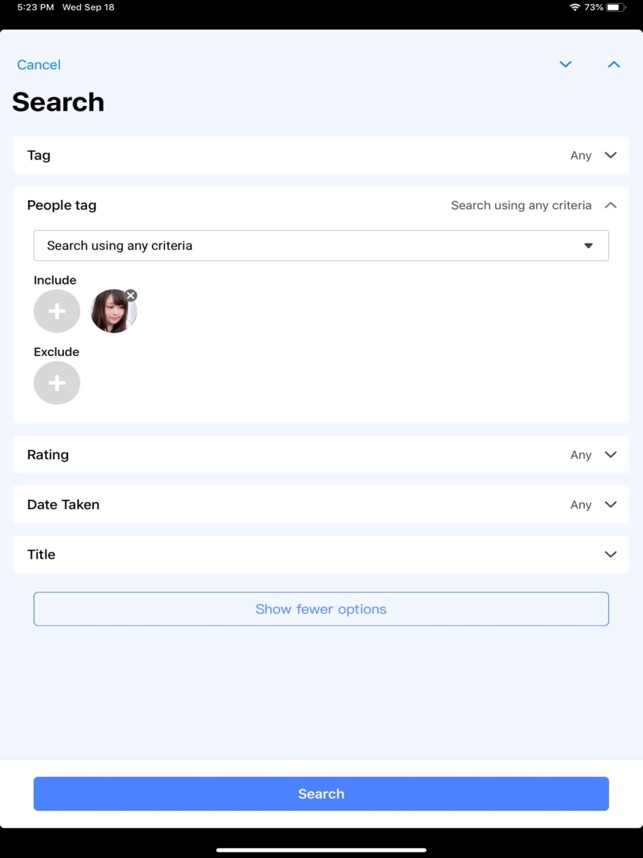Screenshot Description of Search Settings in a Mobile Application:

The screenshot showcases the search settings interface within a mobile or tablet application. 

**Header:**

- At the top, there is a header with a black background and white text. 
- On the top left, the current time is displayed as "5:23 PM" followed by the date "Wednesday, September 18."
- Notably, "Wednesday" is spelled out phonetically as "W-E-D," and "September" is also phonetically misspelled as "S-E-E-P."

**Main Interface:**

- The main section of the webpage starts below the header and has top corners rounded left and right.
- This section has a light blue background.

**Navigation and Main Search Bar:**

- At the top left, there's blue text that reads "Cancel."
- On the top right, there are two blue arrows: an arrow pointing down on the left and an arrow pointing up to the right.
- Below this, aligned to the left, there is large, bolded black text that says "Search."

**Drop-Down Menus and Input Fields:**

1. **Tag Selection:**
    - Beneath the "Search" text, there is a white drop-down menu with rounded corners.
    - The drop-down menu has dark gray text on the left that reads "Tag," and light gray thin text on the right that says "Any" with a dark gray arrow pointing down.

2. **People Tag Selection:**
    - Below the "Tag" drop-down, there's another drop-down that is opened up showing a larger white rectangle.
    - In the top left of this rectangle, bolded black text reads "People tag."
    - On the top right within the rectangle, small light gray text says "search using any criteria" with a dark gray arrow pointing up.

3. **Criteria Selection:**
    - Below the "People tag" section, there is another drop-down menu with a white background and a thin light gray outline.
    - This menu indicates "Search using any criteria" with black text on the left.
    - On the right side of it, a black arrow points down.

**Inclusion and Exclusion Section:**

- Directly under the criteria selection, there are two rows:
   - The top row, labeled "Include" in black text, contains rounded icons.
   - The bottom row, labeled "Exclude," also contains rounded icons under each respective label.

**Additional Options and Action Buttons:**

- Following the inclusion and exclusion sections, there are three more drop-down menus.
- Below these menus, there are two buttons:
   - The first button, positioned on the light blue background, features blue text that says "Show fewer options."
   - The second button is located above a white footer and is a blue button with white text in the center that reads "Search."

Overall, the user interface displays a comprehensive setup for defining and executing search criteria within the application.